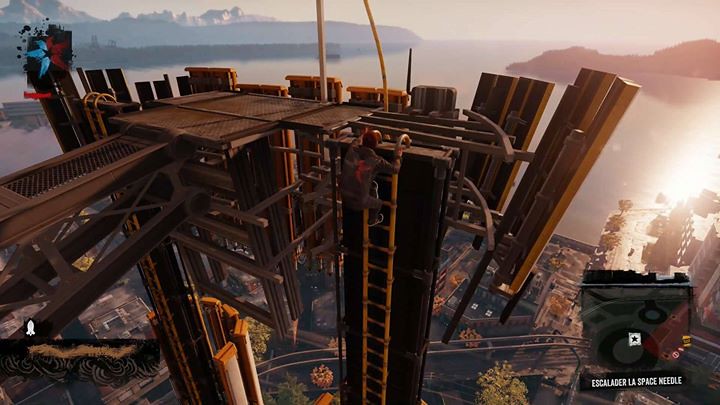Screenshot from a modern 2.5D game showing a player character climbing a yellow ladder on a cell phone tower high above a city. The tower features a steel railing-like scaffolding around it, reinforcing the industrial aesthetic. In the top left corner of the screen, the health bar and player icon are visible, indicating the player’s status. The bottom right corner displays the game UI with a minimap, indicating the current location as "Escalada." The backdrop consists of square yellow antennas, emphasizing the height and the technology-driven environment of the game setting.